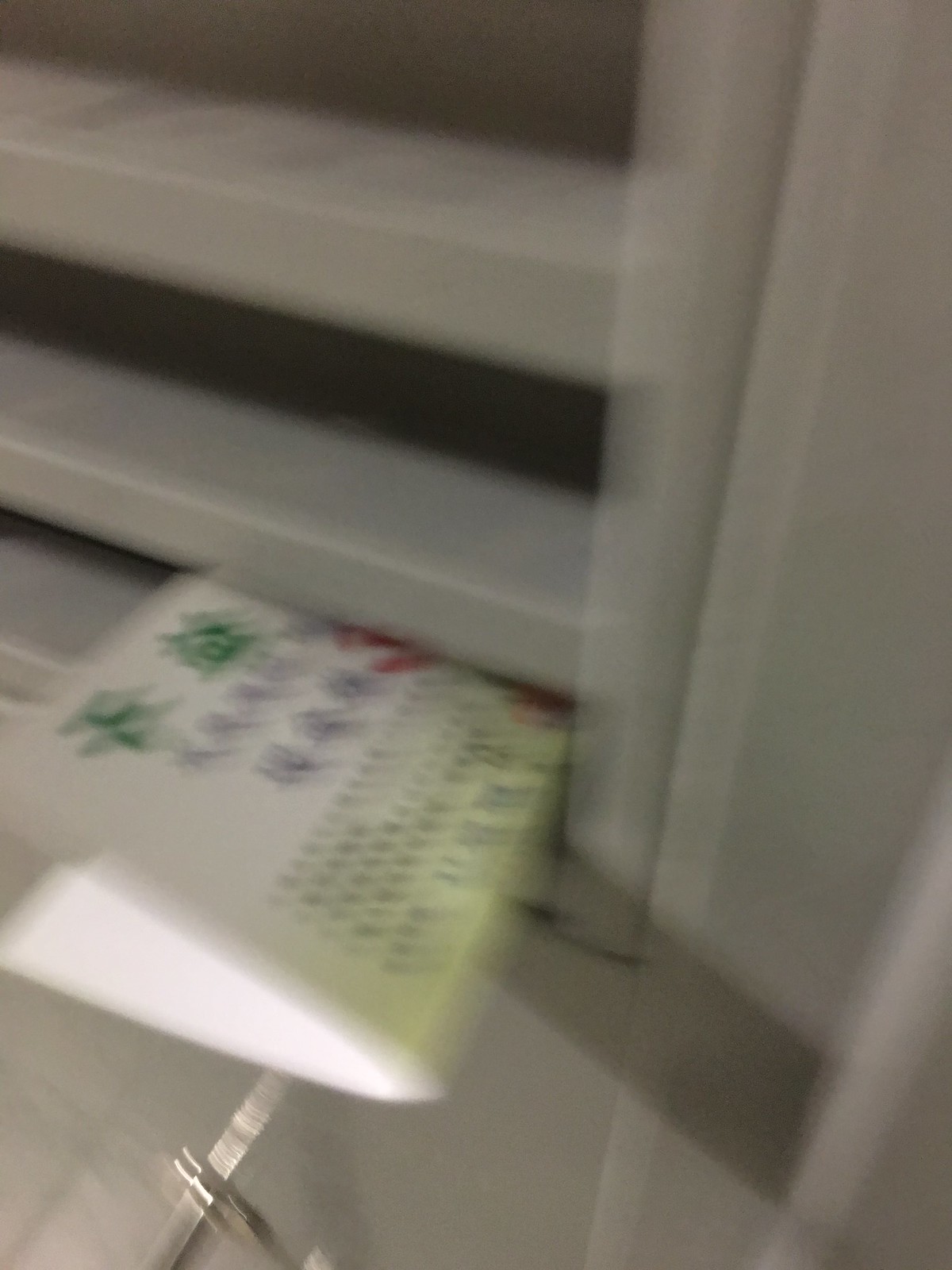The image displays a blurry scene with a white background. Dominant in the frame is an object that appears to have slats, suggesting it might be a window or a similar structure. The overall aesthetic seems slightly dusty. A notable feature in the photo is a folded piece of paper embellished with Asian characters, possibly in green and blue hues. Amidst the blur, there is also an area with smaller Asian text set against a yellow background. This paper is partially inserted between the slats of the main object. Underneath, there seems to be a metal element, though the indistinct quality of the image makes it difficult to identify its exact nature or function. The scene hints at the paper being held or supported by an unseen force or object.